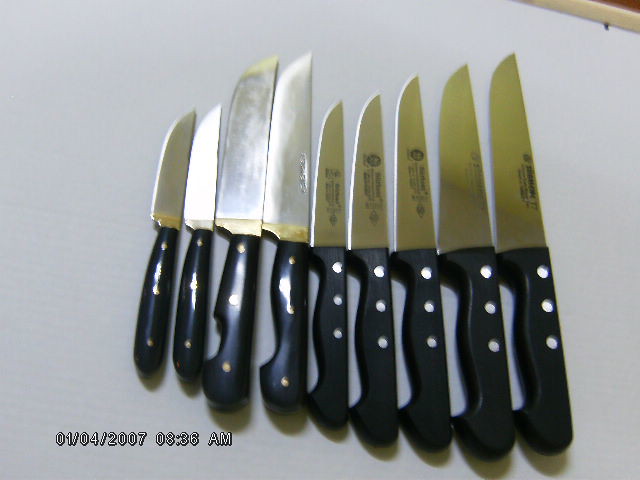The image features a zoomed-in view of nine assorted kitchen knives arranged on a white surface, likely a counter with light brown molding at the edge. A date and time stamp at the bottom of the photo reads "01/04/2007 08:36 AM," indicating it was taken on January 4th, 2007, at 8:36 in the morning. 

The knives, all with black handles, range in type and size from butter knives to more pointed chef's knives suitable for cutting meat. The handles feature rivets, with the first four knives having gold circles and a gold-colored area at the base where the handle meets the blade. The remaining knives have silver rivets and may include short paring knives and one in a cleaver shape. Some of the knives on the right side of the image have blurry text, likely indicating the brand or company name.